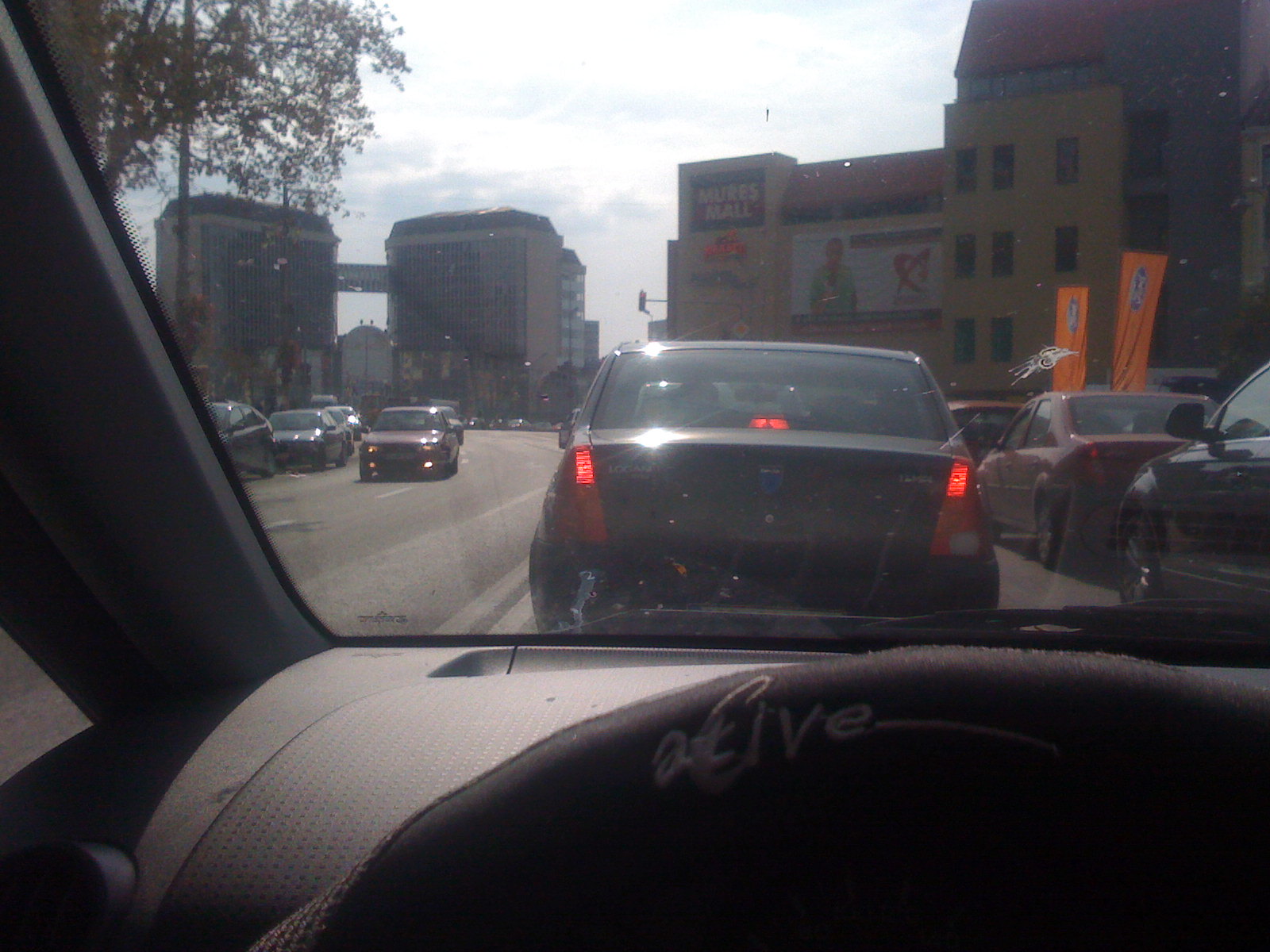A vibrant daytime photograph taken from the driver's seat of an American car captures a bustling city street scene through a slightly dirty windshield. In the foreground, part of the steering wheel is visible, framing the image. Directly ahead, a sedan with all three brake lights illuminated indicates it is either stopped or slowing down. To the left, there's a lane with oncoming traffic, with a row of parked cars alongside the street. The background is dominated by a large multi-story hotel, approximately eight or nine stories high, connected by a bridge spanning between two identical buildings. The pale sky is dotted with light clouds, while a tree's foliage is visible in the upper left corner. To the right of the center, a five or six-story white or off-white building prominently displays the name "Mures Mall" in capital letters, accompanied by other signage and a photograph of a person on a white banner. Orange decorative road flags can be seen just beyond additional parked cars, enhancing the scene's commercial atmosphere. The whole composition captures the vibrancy and architectural elements of the city, with all vehicles and buildings converging towards the Mures Mall.